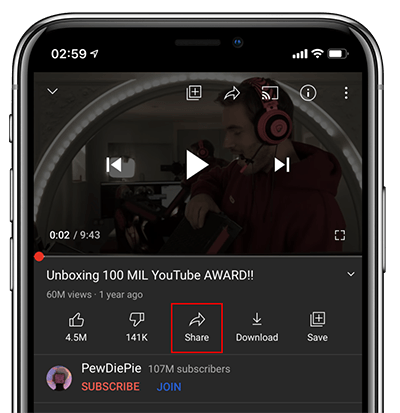This is a detailed photograph showcasing the upper half of a modern metallic black cell phone against a white background. The phone's screen displays a paused video interface. In the upper left corner, the time is shown as "02:59," while the upper right corner features icons representing cell signal bars, Wi-Fi connectivity, and battery status.

Prominently centered on the screen is a play button for video playback, flanked by backward and forward shuffle buttons. The paused video thumbnail reveals an image of a man, identifiable as a white male with dark hair, a beard, and a mustache. He is wearing a red hoodie and red headphones equipped with a microphone.

Beneath the video thumbnail, the playback indicator reads "0:00 / 9:43," indicating that the video duration is 9 minutes and 43 seconds long, yet none of it has been played. Accompanying text reveals the video's title, "Unboxing 100 MIL YouTube Award," which has amassed 60 million views over the past year.

A red box highlighting the share icon is also visible. Below, the publisher's name, "DewDiePie," is written in white font with a subscriber count directly beneath it reading "107 million subscribers." The subscription options are prominently displayed with "Subscribe" in red and "Join" in blue. Despite the familiarity with the creator, there is surprise at his appearance.